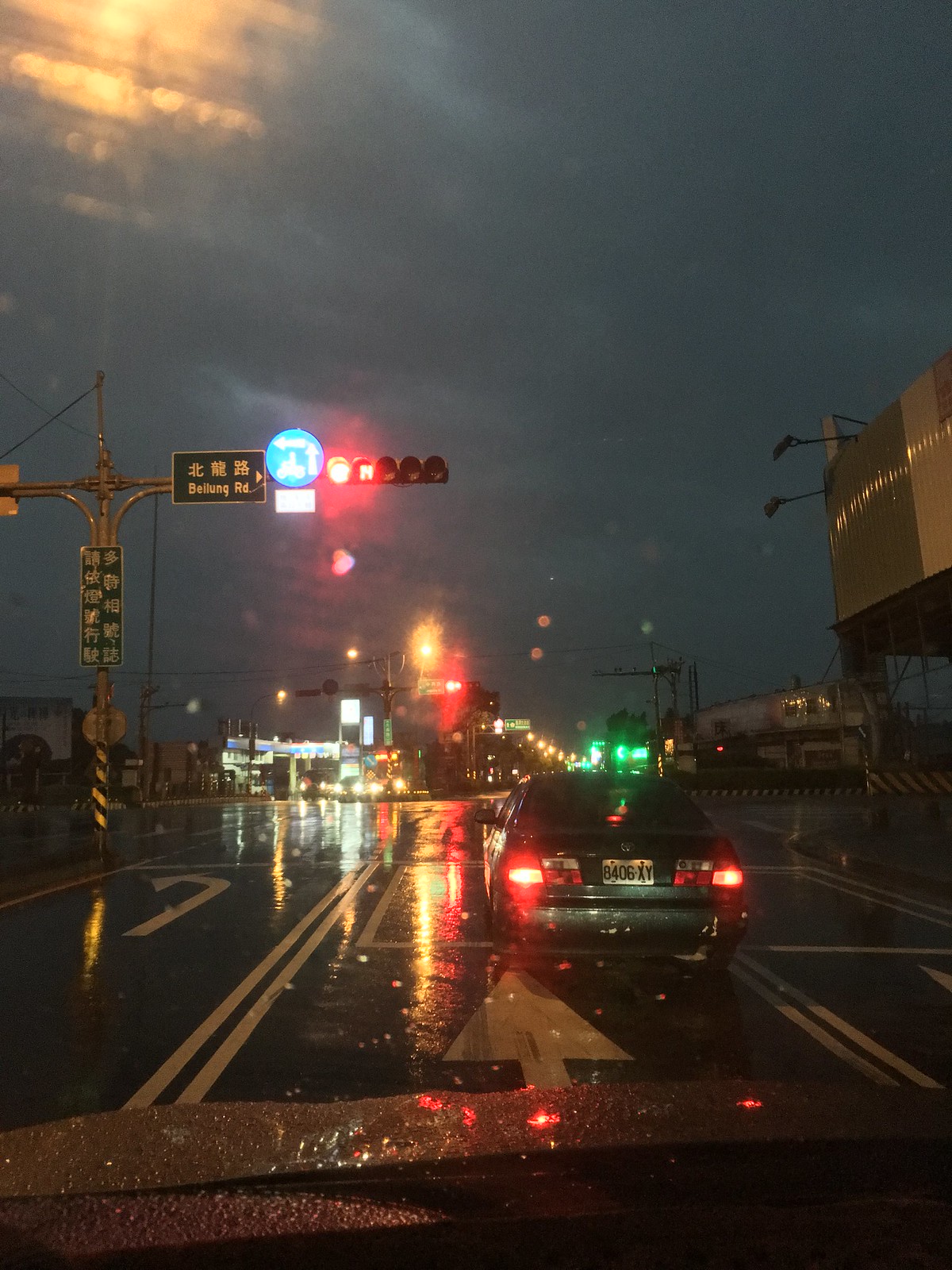This nighttime photo, likely taken in an Asian city such as China or Hong Kong, shows a rain-soaked street glistening under various light sources. The image is captured from the front windshield of a red car, revealing a bustling urban scene. Directly ahead is a dark green sedan with the license plate 8406XY, stopped at a traffic light with its brake lights illuminated. The street features a left turn lane and two straight lanes, mirrored by three lanes in the opposite direction, all separated by a central barrier adorned with streetlights. Above, a traffic light displays red, adding to the vivid reflections on the wet pavement. To the left, a sign indicates "Beijing Road" in both English and what appear to be Chinese characters, while further signs in Oriental script are scattered throughout the scene. The right side of the street includes a mix of buildings, such as shops, a gas station, and possible residential structures, all dimly lit, contributing to the quiet, rainy atmosphere of the urban landscape.